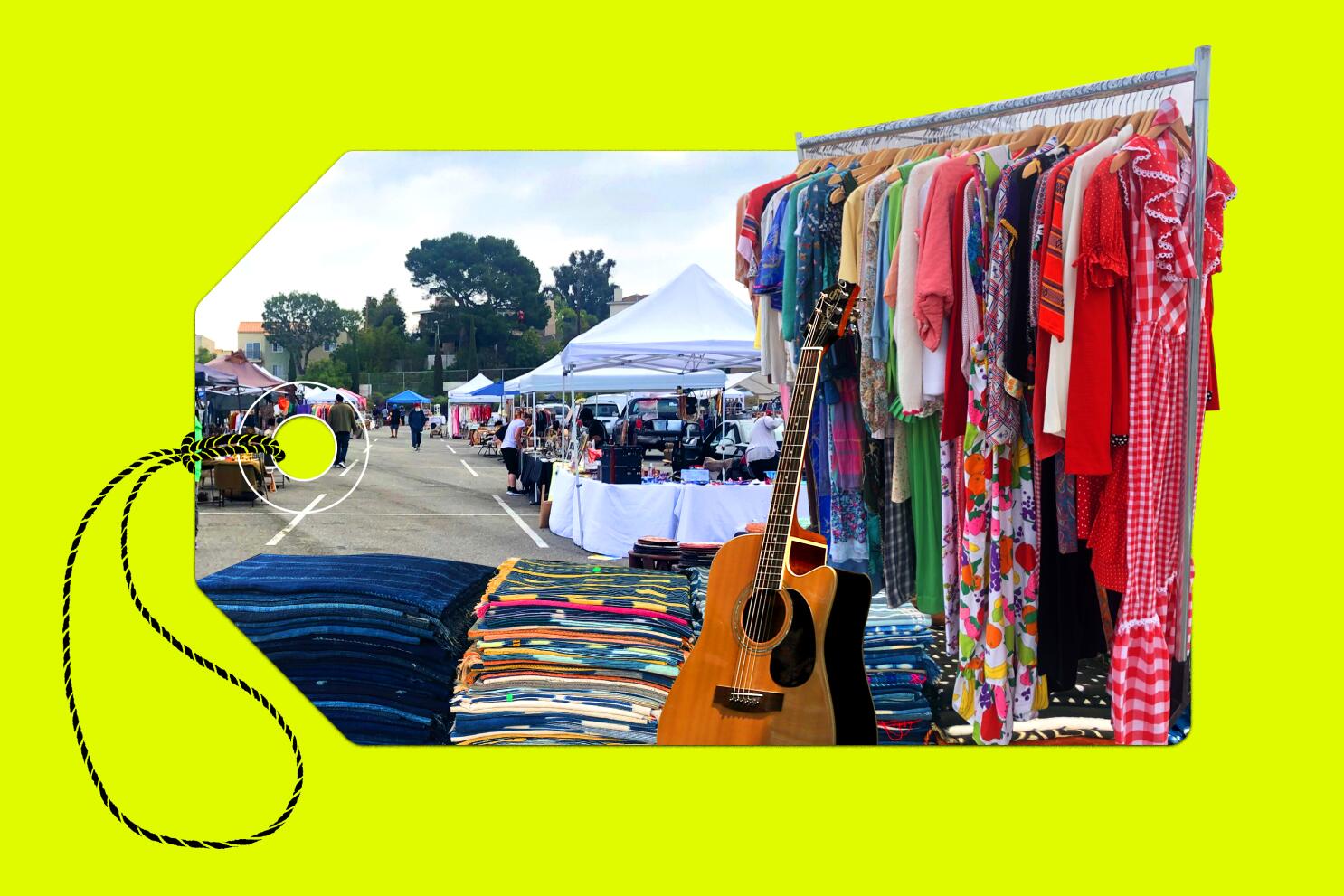The image depicts an outdoor rummage sale set in a parking lot under a clear blue sky. The photograph is shaped like a shopping tag, complete with a hole punched through it on the left. A black-and-yellow string loops around the tag, emphasizing the market-like feel. The background of the image is a yellowish-green hue, creating a vibrant and inviting atmosphere.

Within the tag-shaped photograph, several white and blue canopies are set up, indicating the presence of booths where a variety of items are being sold. People are seen walking around and browsing the assortments of goods. A collection of different colored tapestries is neatly stacked in the foreground, with deep blue ones on the left and multicolored ones to the right. An acoustic guitar is propped up against these tapestries, contributing to the eclectic mix of items on display.

To the right of the guitar, a silver curtain rod serves as a makeshift clothes rack, holding a variety of colorful dresses and shirts, including hues of red, white, green, and blue. Beyond the immediate foreground, the image captures the bustling energy of the sale, with cars parked to the side and people engaging with the sellers under the canopies. Trees and a building provide a backdrop, completing the lively scene of this outdoor event. Various items such as jewelry, clothes, and other trinkets are visible, illustrating the diverse offerings typical of a flea market or yard sale.